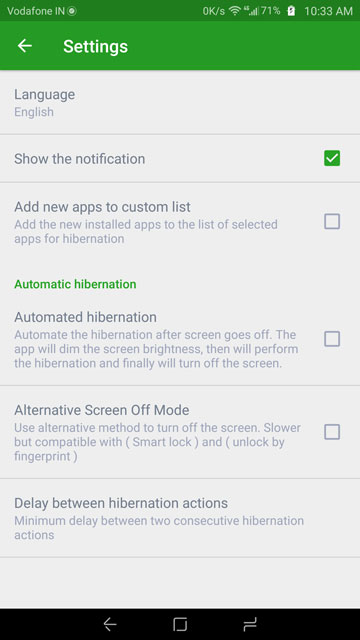Screenshot Description: Detailed Settings Menu on an Android Tablet

The screenshot captures the settings menu on an Android tablet, identified by its wide screen and familiar three-button navigation layout at the bottom. The service provider displayed at the top is Vodafone India (Vodafone IN). The status bar indicates that there is zero kilobytes per second of data transfer at the moment. The tablet is connected to Wi-Fi, has mobile data enabled with a 4G connection, and shows strong signal strength with four out of five bars. The battery level is at 71% and is currently charging. The time displayed is 4:33 a.m.

At the top of the settings menu, a green header with the title "Settings" is prominent. The main language is set to English. Various settings options include:
- "Show notifications" which is enabled.
- "Add new apps to custom list" which, if enabled, would automatically add newly installed apps to the selected apps list for hibernation, is unchecked.

Under the "Automatic Hibernation" section:
- "Automatic hibernation" itself is described as automation that occurs after the screen goes off, where the app will first dim the screen brightness, then perform the hibernation, and finally turn off the screen. This feature is currently unchecked.
- "Alternative screen off mode" is an option to use a slower method to turn off the screen, compatible with Smart Lock and fingerprint unlock, which is also unchecked.
- "Delay between hibernation actions" refers to the minimum delay between two consecutive hibernation processes.

At the bottom, the standard Android navigation buttons are visible:
- The back button.
- The home/menu button.
- The app list button, which allows quick access to recently used applications.

This detailed screenshot encapsulates various configurations available on an Android tablet undergoing settings customization.